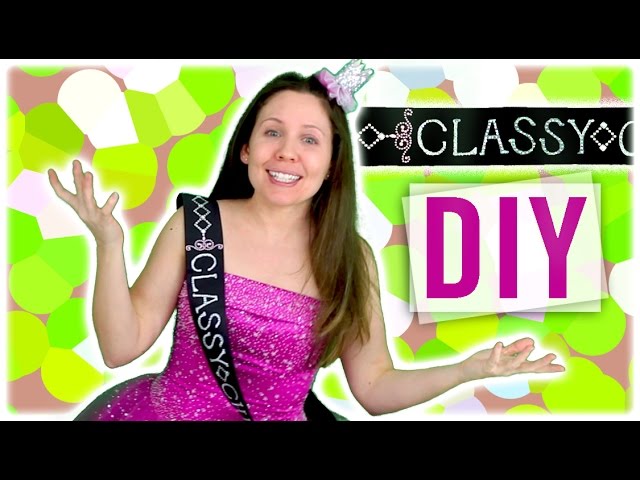The image features a woman in her late 20s or early 30s with long, light brown hair and bluish eyes, smiling playfully with her arms out to her sides as if making a "what" gesture. She is dressed in a sparkly, sleeveless hot pink dress adorned with a pink and silver bow on the left side of her head, and she sports a mini top hat on the right. Draped over her right shoulder is a black sash with white lettering that spells "CLASSY". The background is a vibrant, geometric paper collage consisting of blobs of green, white, lighter green, brown, and blue. The photo is framed with thick black borders at the top and bottom. To the woman’s right, the word "DIY" is displayed prominently on a couple of sheets of paper in tall, purple letters, matching the hue of her dress. Additionally, a black banner with white text that says "Classy" appears in the upper right corner, suggesting this image is from a blog called "Classy DIY."